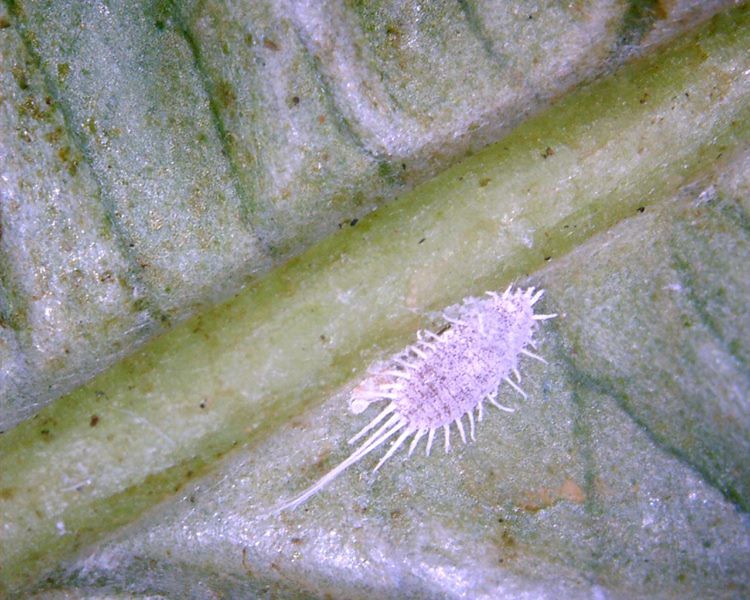The image features a detailed close-up view of a small, lavender-colored bug situated on a vegetation surface that resembles the spine of a leaf. The surrounding area displays two medium-brown rock walls covered with dark to medium green mossy patches. A green seam visually divides the two rock sections, extending from about one-third up the image on the left side to the upper right-hand corner and from the lower left corner to two-thirds up the right side. The bug itself, likely a type of beetle or millipede, is characterized by its oval-shaped body, distinct exoskeleton, and white legs. It has multiple legs encircling its body and a notably long tail that is approximately twice the length of its legs, giving it a double-whipped appearance. The leaf section it rests on has a slight greenish hue, overlaid with a white film, suggesting it might be diseased or unhealthy, enhancing the natural yet rugged setting of this magnified photograph.